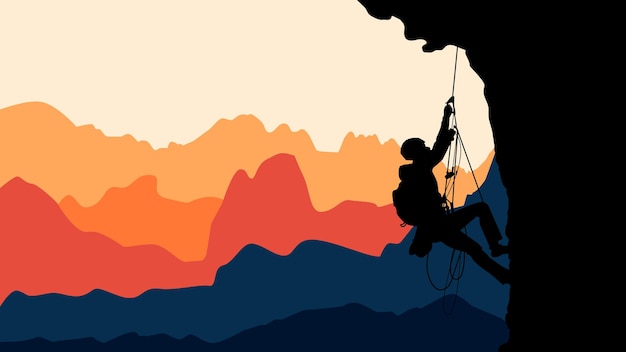This detailed and vibrant art image portrays a silhouette of a climber ascending an overhanging cliff. Both the climber and the cliff are entirely blacked out, emphasizing their dark silhouettes against a rich, multi-colored background. The climber, securely attached with ropes, carries a backpack and wears a helmet, and is portrayed under an overhanging section of the cliff, adding a sense of depth and challenge to the climb. The background is a striking gradient of color, depicting different levels and colors of elevation: craggly blues at the base, transitioning to a spectrum of light blue, rose, peach, and sections of orange that signify various elevations and geological layers. Higher up, the sky shifts from a deep red and dark orange to a lighter peach and ivory hue, culminating in a light pink, creating a dramatic and stylized natural scene that blends realism with a cartoony, computer-generated feel. The overall aesthetic conveys the ruggedness of the mountain landscape contrasted with the simplicity of the silhouetted climber.